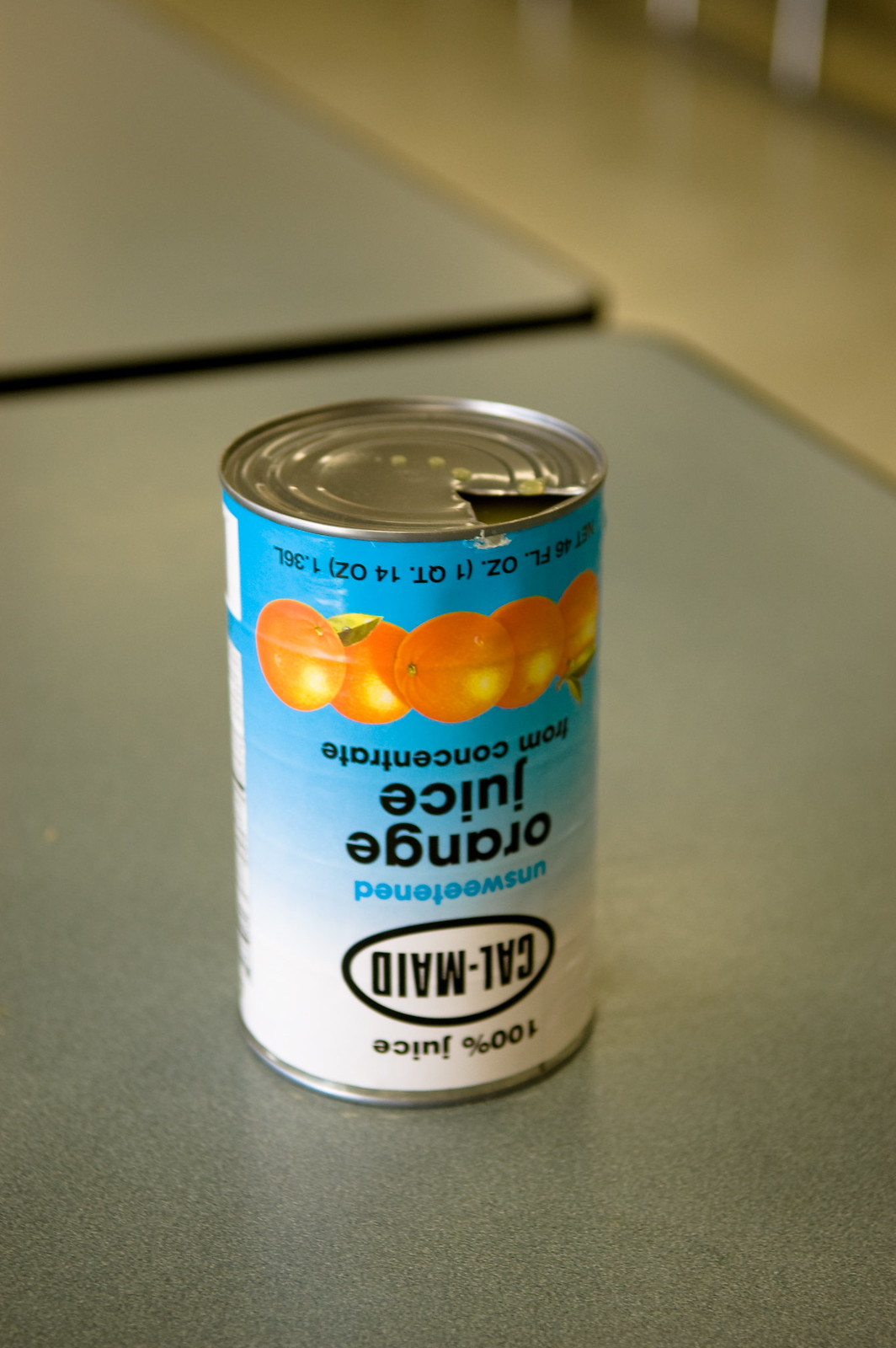In the image, a can of orange juice is prominently featured, positioned upside-down on a gray table. The orientation of the can is evident as the lettering appears inverted. The table extends from the bottom of the image nearly to the top, where the edge of another gray table with a black outer rim is visible, suggesting a cafeteria setting. In the upper right-hand corner, the light brown, tan marble flooring provides a neutral background. The can itself has a white bottom and a blue top due to the angle of the photograph. It is adorned with the phrase "orange juice" and displays five oranges as part of its design. The can's outer rim is trimmed in silver, adding a metallic finish to its appearance.